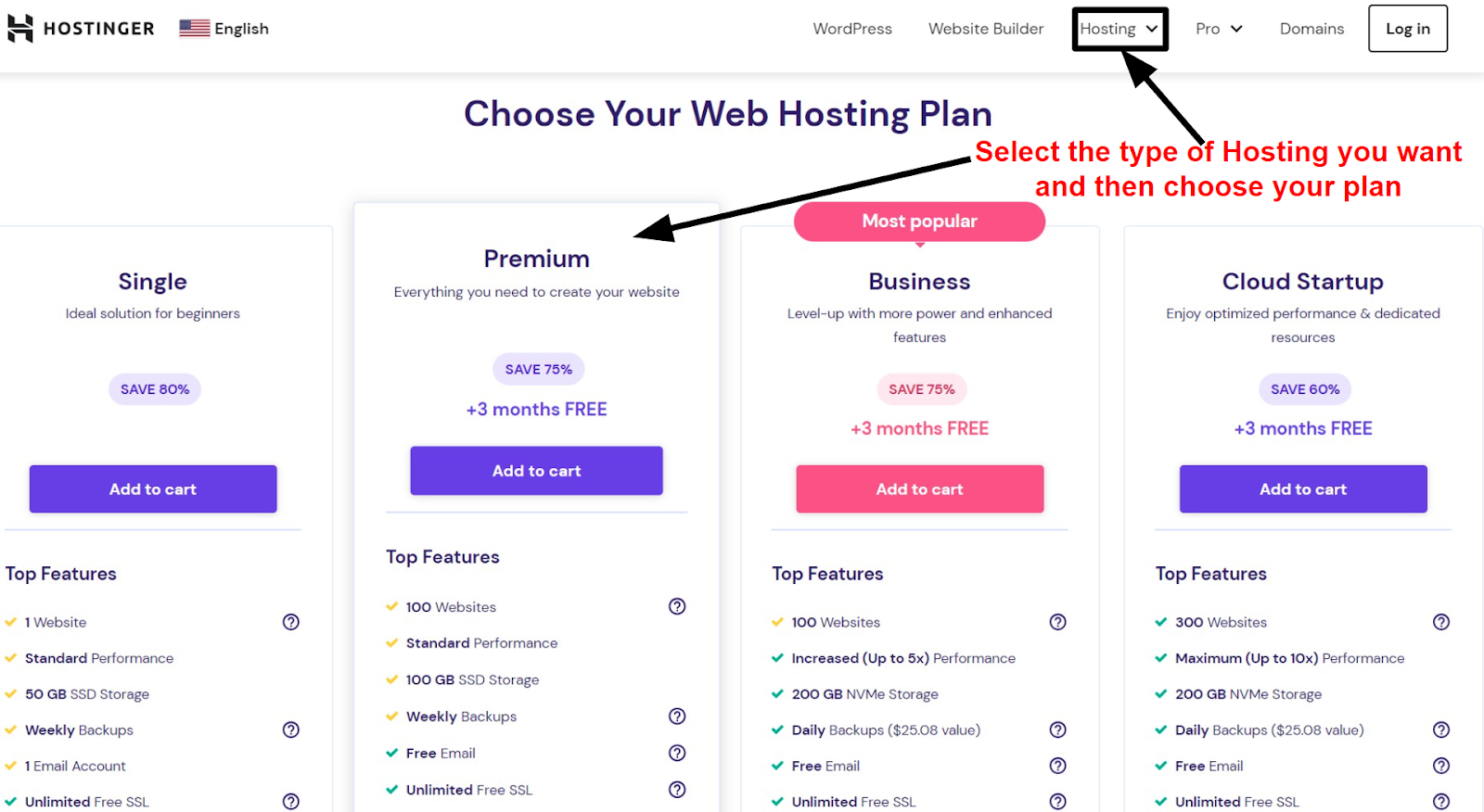This is a screenshot of the Hostinger website. At the very top, the header features the Hostinger logo, an American flag, and a language option indicating English. To the right, there are several navigation links that include WordPress, Website Builder, Hosting, Pro, Domains, and a Login button. The title on the page reads "Choose Your Web Hosting Plan." Below the title, a red banner instructs users to "select the type of hosting you want and then choose your plan."

The page offers four different web hosting plans, each with detailed information and a prominent "add to cart" button in purple or pink. 

1. **Single Hosting**: Advertised as the "ideal solution for beginners," this plan boasts a savings of 80%. There's a purple button beneath it that says "Add to Cart." Key features are listed below the button.
   
2. **Premium Hosting**: Marketed with the slogan "Everything you need to create your website," this plan offers a 75% discount plus three months free. It also features a purple "Add to Cart" button, followed by a list of top features.
   
3. **Business Hosting**: Highlighted as the "most popular" in a pink label, this plan invites users to "level up with more power and enhanced features." It comes with a 75% savings plus an additional three months free. The "Add to Cart" button for this option is pink, and the top features are displayed beneath the button.

4. **Cloud Startup**: Encouraging users to "enjoy optimized performance and dedicated resources," this plan saves 60% plus three months free. It also features a purple "Add to Cart" button and lists the top features below.

Each plan includes a brief description, a significant discount, and a clearly marked button for easy purchase, along with a quick overview of its top features to help users make an informed decision.